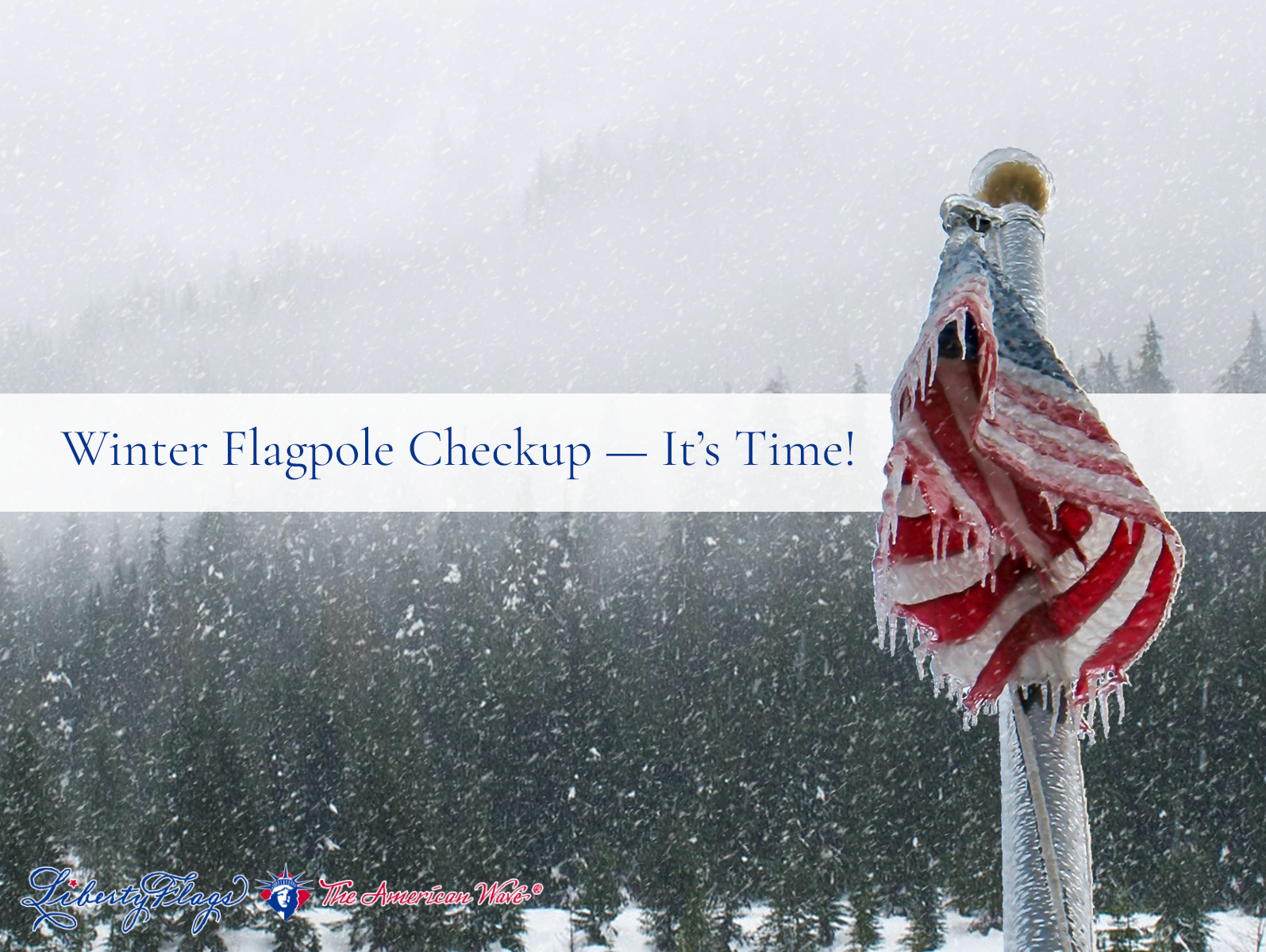In a daytime winter scene, this image portrays a snow-covered American flag on a flagpole, encrusted with icicles hanging down like stalactites, set against a misty, foggy backdrop of pine trees dusted with snow. The text in the center reads, "Winter Flagpole Checkup - It's Time!" accompanied by the Liberty Flags logo, featuring the blue head of the Statue of Liberty against a red square, and the words "Liberty Flags, The American Wave" in red and blue text with a trademark symbol. The image, which appears to be photoshopped together, serves as a reminder for people to take their flags down during the winter to prevent them from freezing on the poles.